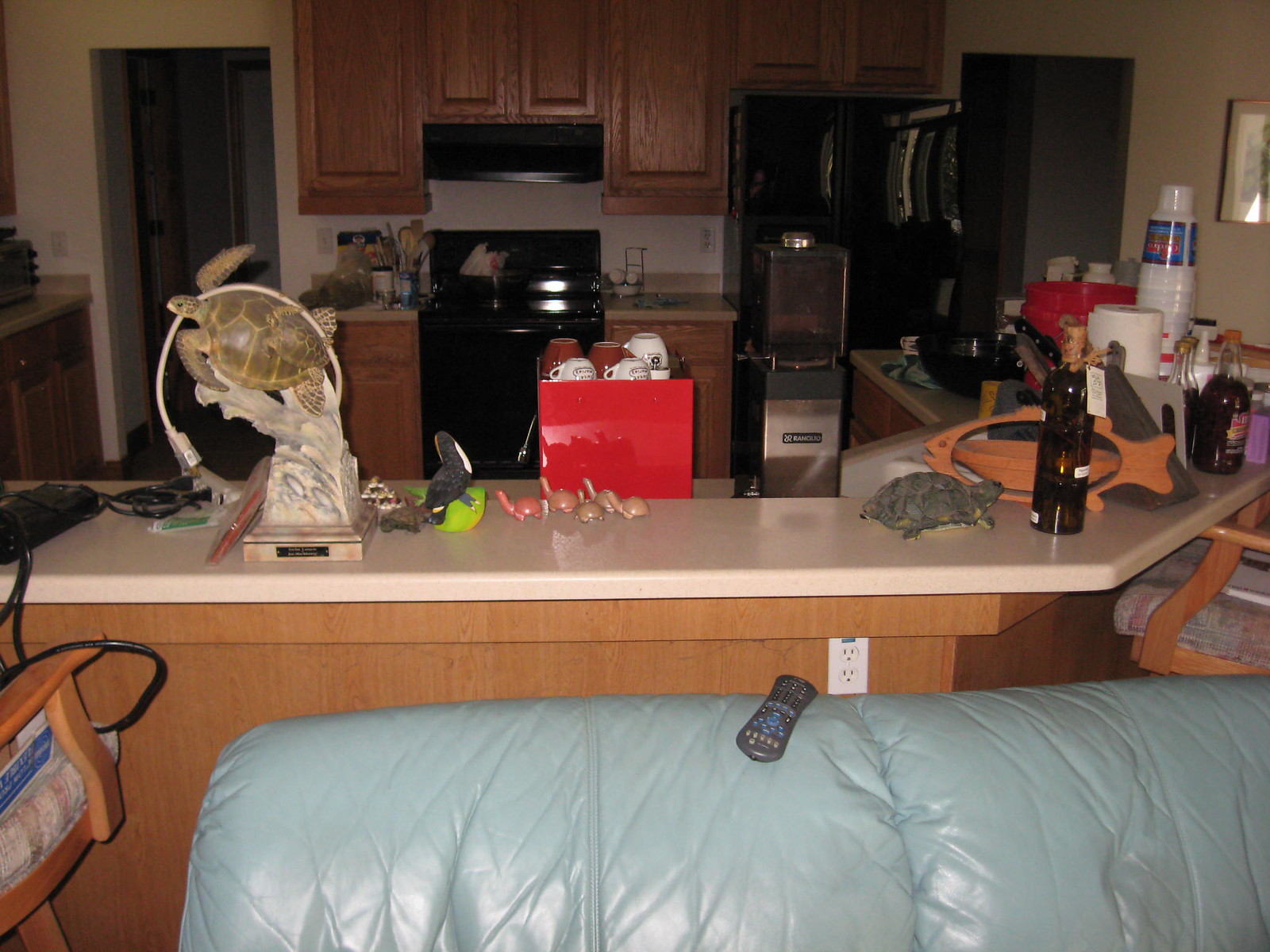In the dimly lit kitchen scene, the foreground features the upper back of a very pale blue leather or pleather couch, on which a black TV remote rests. Just beyond the couch, the cream-colored laminate kitchen counter is cluttered with various items. Several small plastic turtles and what appears to be a real turtle are scattered on the counter, next to a brown glass bottle with a cork and a price tag. 

A wooden fish-shaped design, with an open body that holds a bowl, sits nearby. A red cardboard box topped with several coffee mugs is also visible on the counter. Additionally, there's a trophy-like object featuring a large gray and white wave with a mother turtle and her baby attached to it, draped with a white cord.

The background showcases kitchen cabinets above and below a black stove. The counter is strewn with an assortment of items, including a stack of large plastic drink cups. The sink is visibly full of pots, pans, and dishes. Wooden-frame chairs with light gray and pink patterned seat cushions are pulled up to the counter, completing the scene.